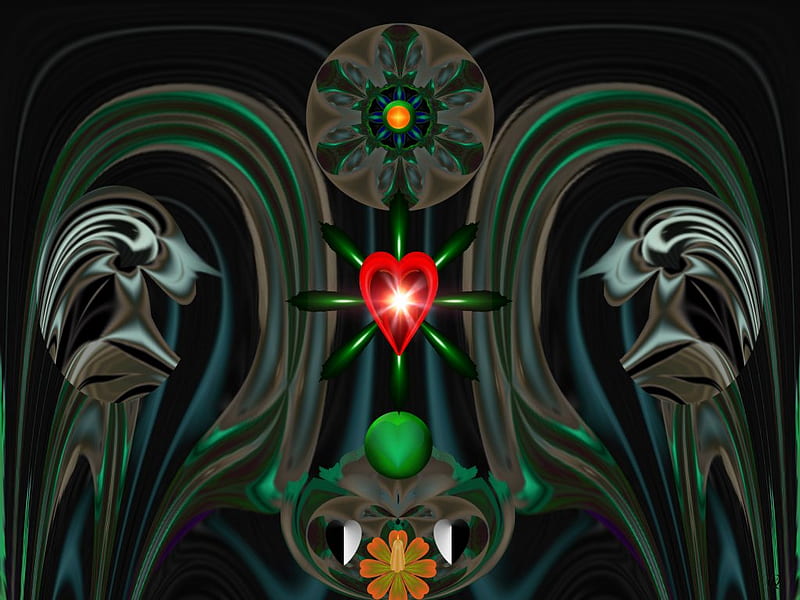The image presents a highly symmetrical and psychedelic computer-generated design set against a completely black background. Central to the composition is a red heart with a bright, yellowish-white starburst at its center, emitting light outward. Surrounding the heart are eight dark neon green lines, resembling stubby posts, positioned in a radial pattern. At the top, there is a circle with intricate detailing: it features brown lobes and a central orange and green motif, giving it a floral appearance with additional layers of turquoise-blue petals.

On either side of the heart, symmetrical silver, metallic figures of women with pointy noses face each other. Their mouths are open, and they exhibit strands of hair that flow backward in gray and black hues, enhancing the mirrored effect. Below the heart, there's a green, apple-shaped form, more blob-like than circular, followed by an orange flower with petals that transition to dark green at their bases.

At the very bottom of the image, white fang-like shapes emerge alongside another flower marked by orange petals and a greenish central section. Additionally, black and white heart emblems are situated to the left and right of the central heart, complementing the overall motif. The entire scene is layered with various hues of green and gray, further contributing to its surreal and dreamy quality.